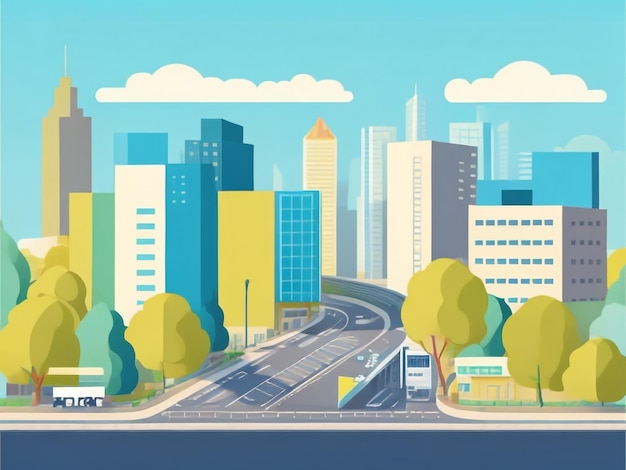The image depicts a vibrant, cartoon-style cityscape with a distinctly animated appearance. Dominating the scene is a divided highway curving to the left, which is devoid of cars but connects to a black roadway at the bottom. The city skyline features an array of towering skyscrapers in hues of yellow, blue, white, orange, avocado green, and darker blue, showcasing a variety of architectural styles. The sky overhead is a clear light blue, adorned with two clouds, one on the left and one on the right, suggesting a tranquil day. In the foreground, tall, lollipop-styled trees line both sides of the roads, adding a whimsical touch. There are street lamps dotting the scene and a bus stop situated at the bottom left, contributing to the urban setting. The overall aesthetic hints at a computer-generated image with some elements appearing slightly distorted or artifacted, giving it a polished yet slightly imperfect look typical of corporate art style illustrations.